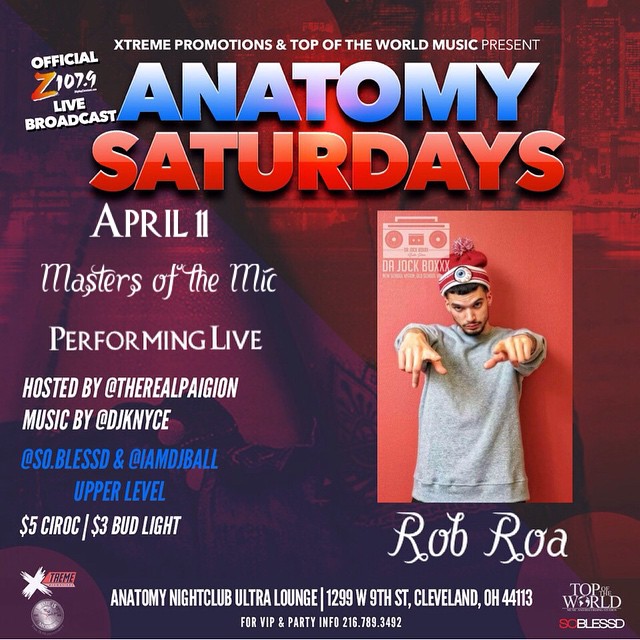This promotional poster for a music event features a tall rectangular design with a red and purple tinted cityscape background. At the top, in bold white uppercase letters, it reads "Extreme Promotions and Top of the World Music Present." Below this, "Anatomy" is displayed prominently in large blue gradient letters, with "Saturdays" in red gradient letters underneath.

The central section includes a tall rectangular photograph of a man, visible from the torso up, pointing forward. He is leaning against a red wall, wearing a gray sweater, a red hat with a red and white pom-pom, and has light skin, a brown beard, and brown hair. The name "Rob Roa" is written in cursive white letters near the photograph.

Further text reveals additional event details: "Official Z107.9 Live Broadcast," "April 11th," "Masters of the Mic Performing Live," and "Hosted by @TheRealPaga." Music will be provided by "@DJNice," "@SoBlessed," and "@IMDJBall Upper Level". Beverage prices are also listed: "$5 Ciroc" and "$3 Bud Light."

At the bottom, the venue is identified as "Anatomy Nightclub Ultra Lounge, 1299 W 9th Street, Cleveland, OH 44113," along with a contact number for VIP and party information: "Call 216-789-3492."